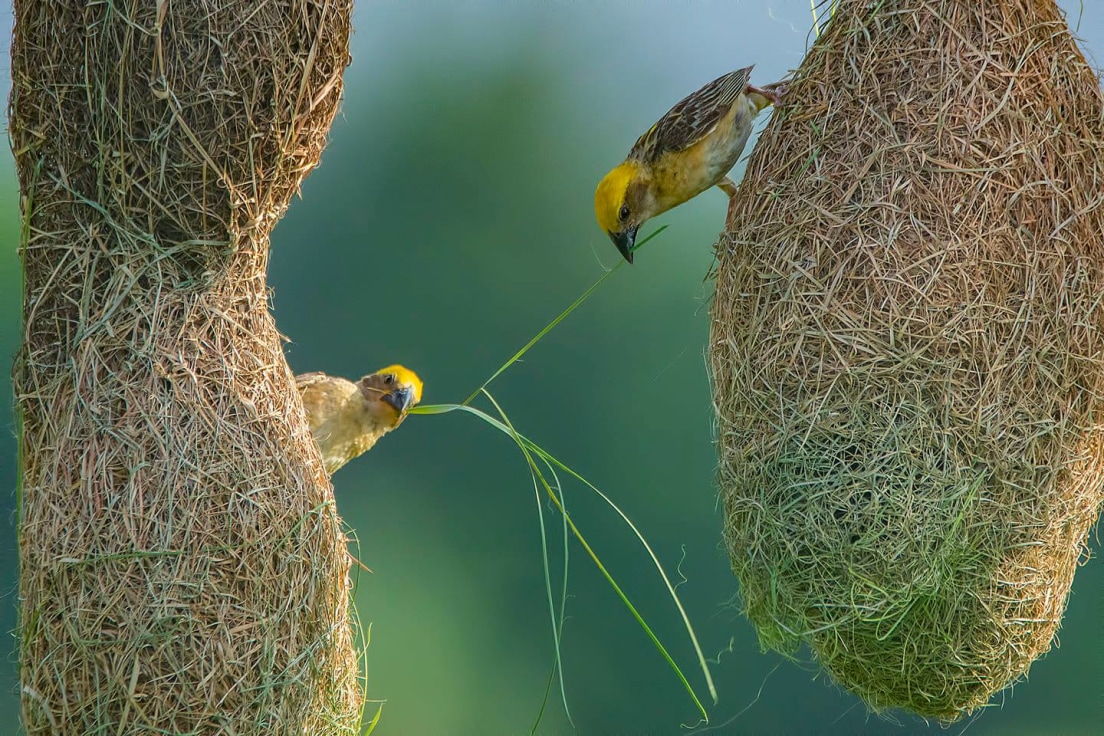The photograph features two small yellow birds with black beaks, perched on dried, beige-colored hay structures. These hay structures, appearing to hang from tree branches, resemble intricately woven nests. The birds, similar in size to finches or chickadees, exhibit bright yellow heads and chests, alongside brown and white wings. Both birds are engaged in the process of nest-building, each grasping a long, vibrant green blade of grass. The bird on the left holds one end of the grass while the bird on the right tugs at the other, seemingly ripping it apart. The scene is set against a sunny backdrop with blurred trees, casting a natural and serene atmosphere. The birds’ positioning is somewhat awkward, with one bird’s head jutting out sideways and the other seemingly hanging upside down, adding a dynamic and animated quality to the image.